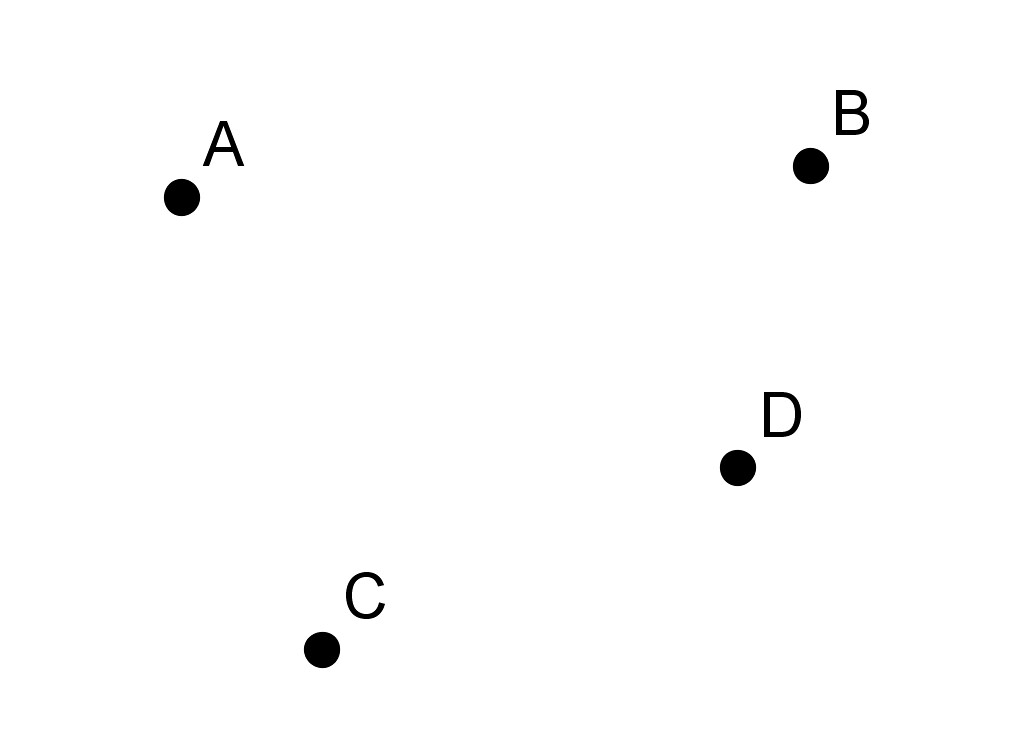The image showcases four black dots on a white background, each labeled with a capital letter. The dot labeled "A" is situated in the upper left-hand corner. Directly across from "A" on the upper right side, slightly higher than "A," is the dot labeled "B." Both labels are positioned to the upper right of their respective dots. Moving down the screen approximately two-thirds of the way and slightly to the right, you'll find the dot labeled "D." Lastly, the dot labeled "C" is located near the bottom, slightly diagonal from "D" and not as far to the left as "A." The labels "A," "B," "C," and "D" are all placed to the upper right of their corresponding dots, creating a visually distinct arrangement across the image.